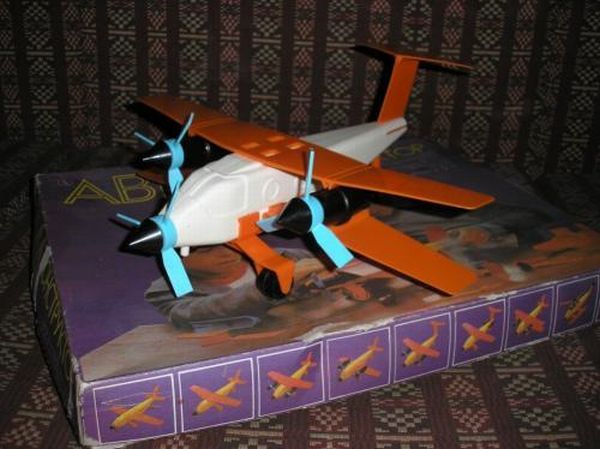In the image, a small model airplane is prominently featured, resting on top of its original purple packaging box. The background is composed of a piece of furniture, likely a sofa or chair, which has an intricate pattern of vertical black stripes interspersed with diamond shapes, in black and gray hues. The model airplane itself has a white body with striking orange wings, and orange accents on the top and rear sections. The propellers are a vibrant light blue, and the landing wheels are deployed as the airplane sits on the box. There are sharp, black pointed tips at some parts of the plane. The purple box below shows the airplane model fully assembled in eight repeated images along the sides, although the plane depicted on the box has a yellow body. Above these images, yellow letters "A" and "B" are visible in the top right corner of the box. The setting appears to be within a home, possibly indicating that someone, perhaps a child in a gray shirt, has been assembling or playing with the model near a table.